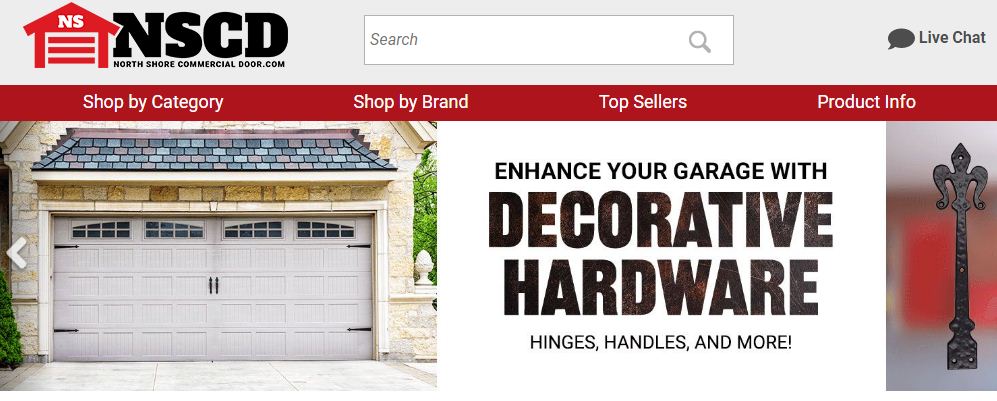This horizontal screenshot features a website banner for North Shore Commercial Door's online store. The image appears clipped, making it exceptionally wide and short. At the very top, a light gray banner displays the North Shore Commercial Door logo, which consists of a red house symbol with the letters "NS" on it. To the right of the logo, the text reads "NSCD, NorthShoreCommercialDoor.com." Centered within this banner is a white search box, and a live chat icon is positioned at the upper right corner.

Beneath the gray banner is a thinner red banner showcasing four headings in white text: "Shop by Category," "Shop by Brand," "Top Sellers," and "Product Info." Below this, a large photograph displays a garage door set against a stone house with a multicolored gray roof. To the left of the photograph, a left arrow button is visible, suggesting navigation options.

Adjacent to the photograph, in large text, the words "Decorative Hardware" are prominently displayed. Above this, smaller text reads "Enhance Your Garage with," and below it, "Hinges, Handles and More." Collectively, the text forms the phrase: "Enhance Your Garage with Decorative Hardware, Hinges, Handles and More."

To the right of this text, set against a blurred red, brown, and gray background, is an intricate piece of decorative metal resembling the top of a metal gate, possibly evoking the design of a fire poker.